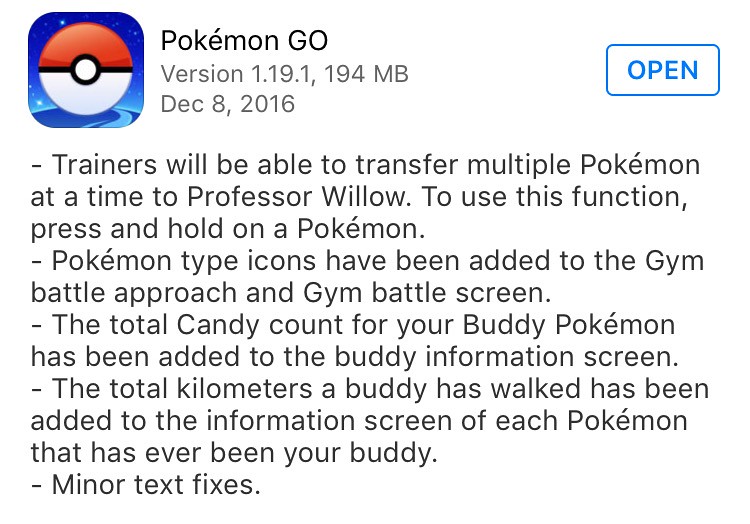The image is a landscape-oriented screenshot displaying patch notes for the mobile game Pokemon Go. In the upper left corner, there is the app's icon, featuring a Pokeball on a blue sky and wavy road background. A Pokeball is a round object with a red top, white bottom, and a central horizontal line separating the two colors, featuring a white dot encompassed by a black border. To the right of the icon, the text reads "Pokemon Go version 1.19.1, 194MB," with the release date "December 8, 2016" positioned beneath. At the top right is a blue "OPEN" button inside a rectangular outline. Below, a list details the changes in this update: trainers can transfer multiple Pokemon at a time to Professor Willow by pressing and holding on a Pokemon, Pokemon type icons have been added to the gym battle approach and battle screens, the total candy count for your buddy Pokemon is now displayed on the buddy information screen, the total kilometers a buddy has walked is now shown on the information screen for each buddy Pokemon, and there have been minor text fixes.